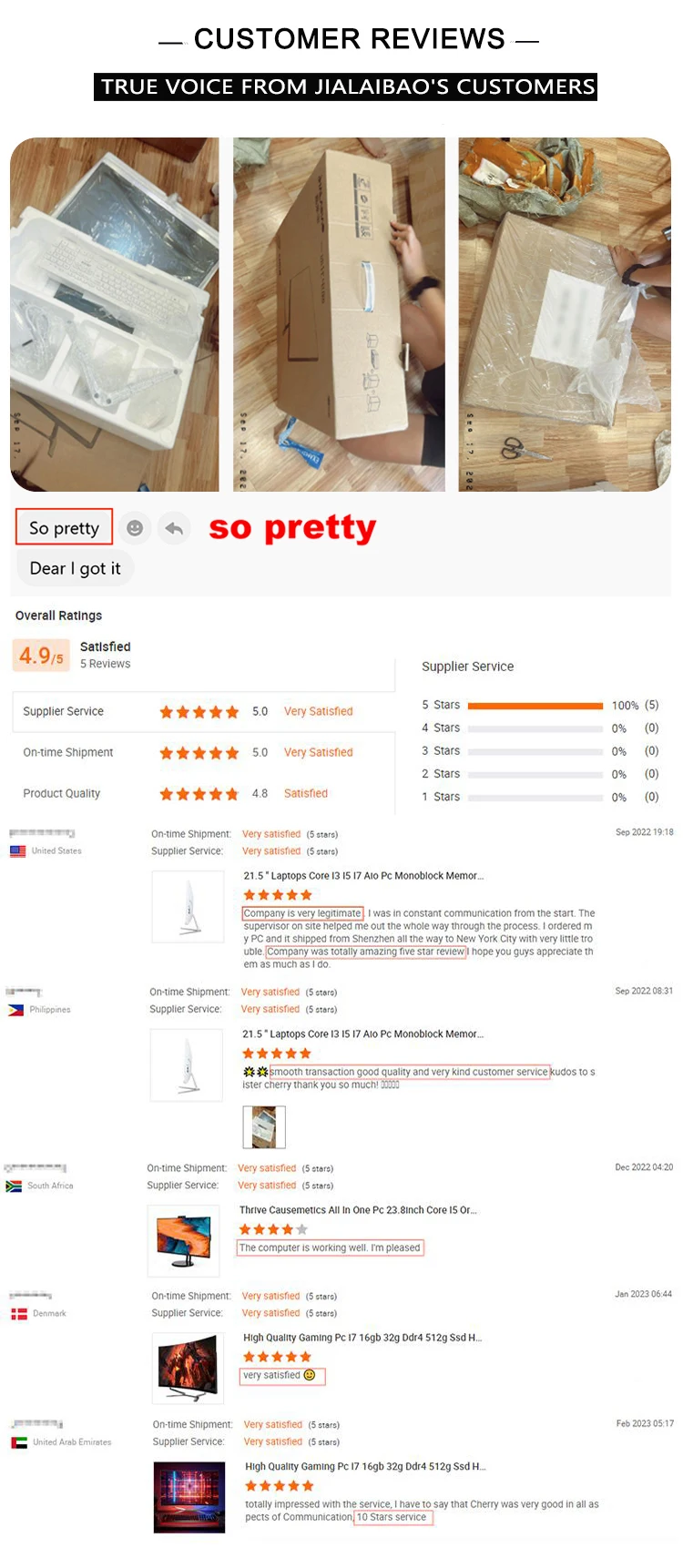The image depicts a section of a website dedicated to customer reviews. The background is entirely white. At the top of the section, there is a thin horizontal line, followed by the heading "CUSTOMER REVIEWS" in bold, black, capital letters. Another line appears right after the "S."

Below this heading, there is a black rectangular section that contains white text stating "TO VOICE FROM," followed by "JIALAIBAO'S" in white text with an apostrophe. Further down, the section shows three different images. Below these images, there is a bold, red-bordered box with the text "so pretty" inside, written in lowercase, bold red letters.

The subsequent line reads "Dare, I Got It" and highlights an overall rating of 4.9 out of 5, based on satisfied reviews from five reviewers. The reviews for supplier service are detailed as follows:
- Supplier Services: 5.0 stars, very satisfied.
- On-time Shipment: 5 stars, very satisfied.
- Product Quality: 4.8 stars, satisfied.

The website further displays reviews from the United States, the Philippines, South Africa, Denmark, and the United Arab Emirates. The email addresses or usernames of the reviewers are blurred out for privacy purposes. The dates when the reviews were posted are also provided.